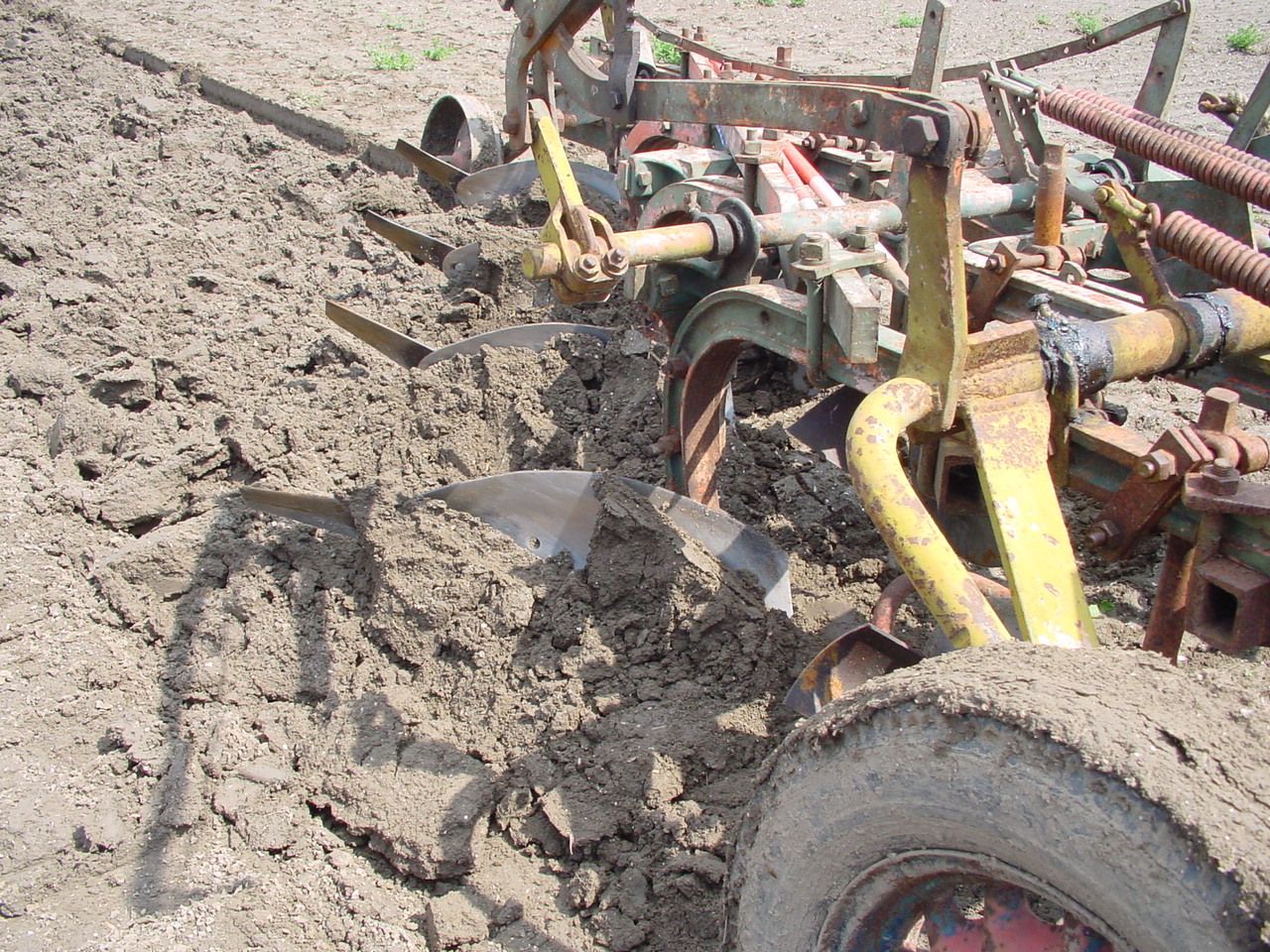This image features a close-up view of a plow attachment connected to a tractor, engaged in tilling a field. The central focus is on the plowing tool, its blades actively breaking up the light brown, flaky soil which appears fertile and sandy rather than clay-like. The plow has four rotating blades, partially embedded in the earth, efficiently churning up the top layer. In the image, metallic components including multiple rusty springs and several areas with gray weld marks, indicating previous repairs, are visible. The metal parts originally painted in yellows, reds, and greens now appear faded and rusty. The device's tires, especially one prominent tire in the bottom right corner, are caked with mud and display some red and blue coloration. In the distant background, a few patches of grass dot the otherwise barren field. The scene suggests a piece of old, well-worn farming equipment actively in use, likely being pulled by an unseen tractor to prepare the land for cultivation.